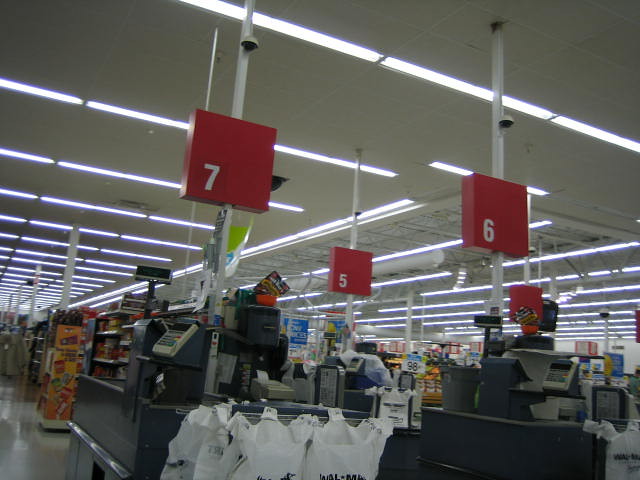This image portrays the interior of what appears to be a Target store, viewed from a low angle near the checkout area. Dominating the scene are several red signs hanging from the ceiling, clearly marking checkout lanes 5, 6, and 7, with large white numerals on the red backgrounds. The focal point at the bottom of the image includes a cluster of plastic shopping bags positioned at the registers. To the left of the register, a credit card reader is visible, while to the right, another aisle can be discerned. The ceiling is lined with extensive track lighting, illuminating the depth of the store, though the overall image leaves much of the store’s layout to the imagination due to the angle of the shot.